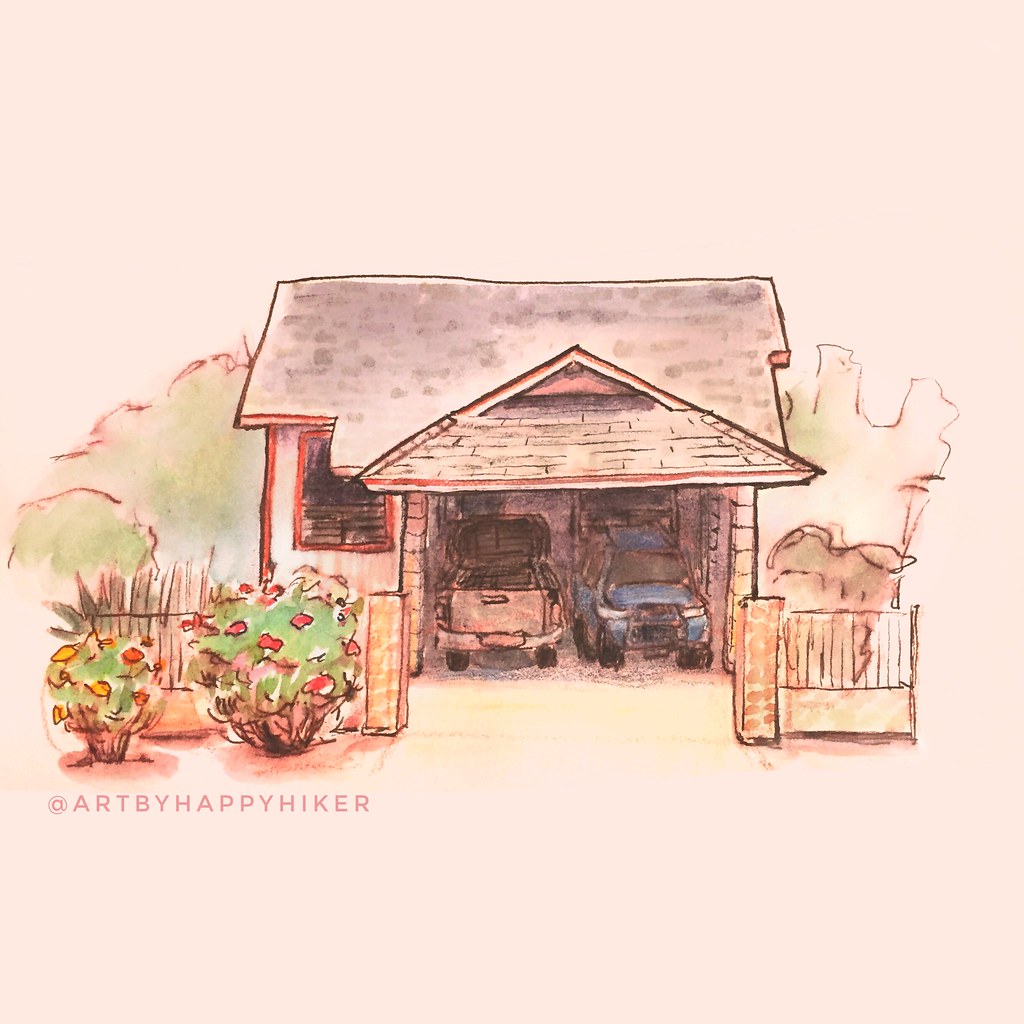This image, titled "Art by Happy Hiker," is a detailed watercolor painting of a charming small cottage. The house features a distinct pink roof with subtle gray and deep pink dots, adding texture. A single window is present on the left side of the house. The open garage shows two vehicles parked inside: on the left, a faded pale yellow truck with a silver bumper facing forward, and next to it, a blue SUV with silver headlights. In front of the house, a brown fence encloses the small front yard adorned with various shrubs and plants. To the left of the driveway entrance outside the gate, there are two prominent shrubs: a smaller yellow shrub and a larger green shrub with red flowers. Additionally, the lower left corner of the painting contains a sign reading "Art by Happy Hiker," emphasizing the work's artistic origins. The grassy front yard is highlighted by shrubbery and trees, loosely sketched and colored in an abstract manner, adding a dynamic and slightly whimsical element to the piece.